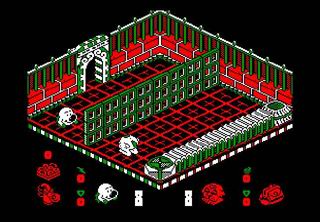The image depicts a screenshot from an old video game with an isometric perspective. The scene is set in a saloon-like room that features a heavily stylized red and green color scheme. The room has a tile floor patterned with red and black stripes, and there are intricate symbols in the center. The walls are predominantly green, decorated with white-bordered squares and large sections that resemble shelves or countertops. A green and white doorway is prominently featured, and to its left, there appears to be a face-like design, possibly of a dog. In the middle of the room, a grating separates two players who each have the number 8 displayed next to them. They appear to be either competing or cooperating in this setting. Various red, green, and white icons are visible at the bottom of the screen, suggesting gameplay elements related to positioning or stacking items on a grid. The entire scene is set against a black background, adding to its distinctive appearance.